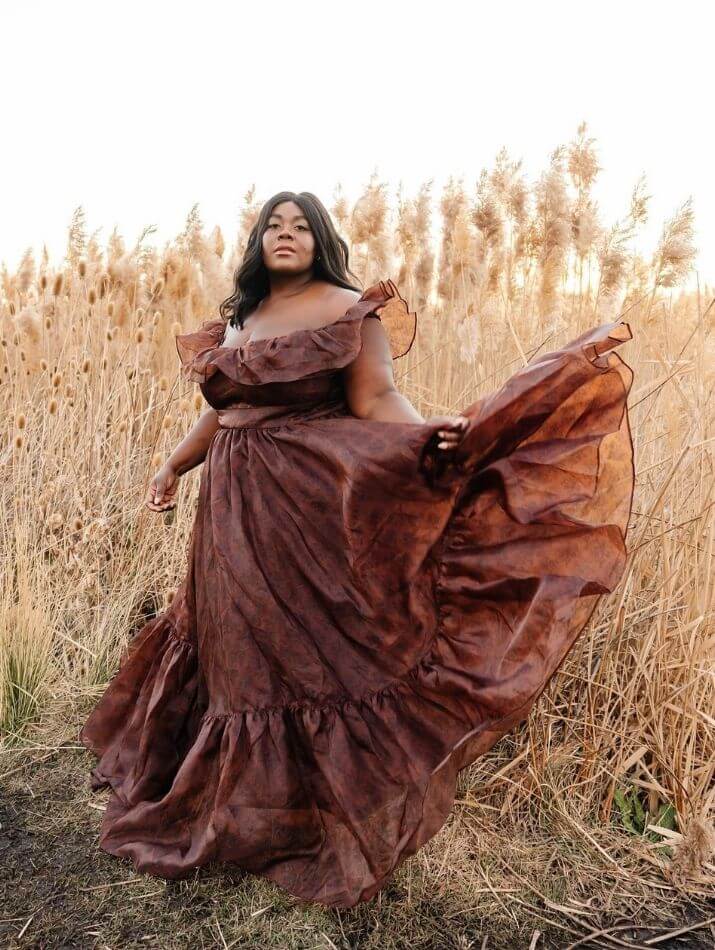In this outdoor photograph taken in natural light on a clear day, a heavyset black woman with long, shoulder-length black hair gazes directly into the camera, her expression serious and composed. She is elegantly dressed in a full-length, dark brown, sleeveless gown that flows luxuriously down to the ground and spreads out around her. The dress has a frilly top that exposes her arms and the upper part of her chest. She holds up the right side of the dress, causing it to ripple slightly as if caught by a gentle breeze, showcasing its flowing nature. The setting is a striking contrast of textures, with the woman standing on a patch of short, manicured grass in front of an expansive field of tall, dry, golden wheat, creating a dramatic and picturesque backdrop. There is no jewelry adorning her, and her right hand is unobstructed. The photograph appears professionally taken, possibly intended to highlight the elegance and design of the dress.